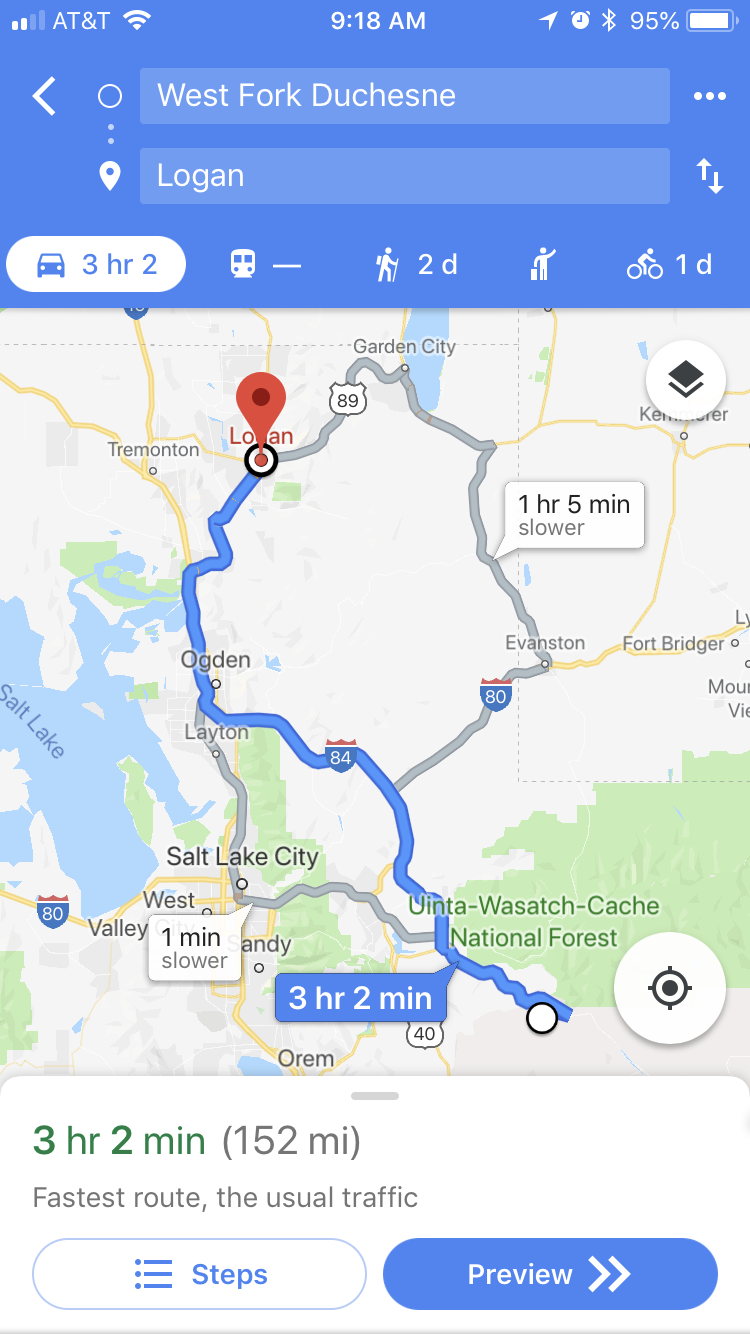The image displays a smartphone screen showing a map with a detailed route from West Fork, Duchesne, to Logan. The phone has 95% battery life, and the time displayed is 9:18 a.m. The network provider is AT&T, and there is an active internet connection. At the top of the screen, the search bar shows "West Fork, Duchesne" and below it, another search bar displays "Logan," indicating a travel route from one location to the other.

The travel information reveals it takes three hours and two minutes by car to cover the 152-mile distance, with the driving time highlighted in green. Alternative transportation options are also noted: walking takes two days, and biking takes one day. There is an icon for a taxi, but no information is provided next to it.

The map itself is visible below these details, showing a route marked with a red pin from the starting point to the destination. Additional options on the screen include a blue circle labeled "Preview" with two right-facing arrows, and another circle for "Steps." The caption emphasizes that the route is the fastest one available, given the usual traffic conditions.